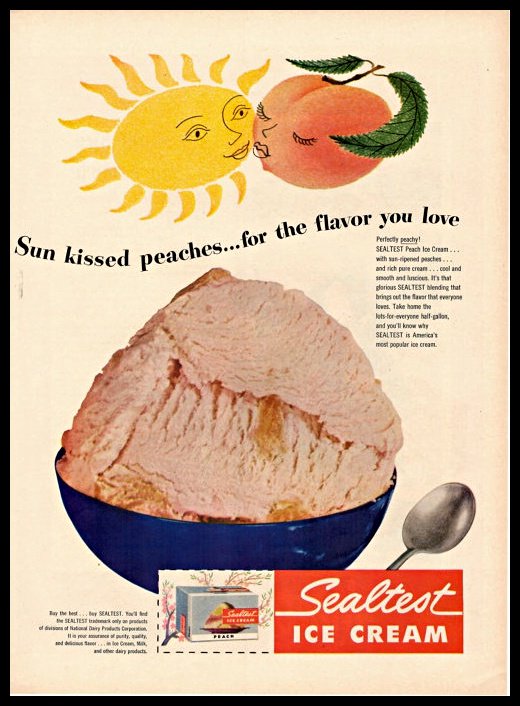The image is an advertisement for Sealtest ice cream, framed with a black border and featuring an aged white background that gives it a vintage feel, possibly from the 1950s or 60s. At the top of the ad, there is a charming cartoon scene where a yellow sun, depicted as a woman with bright radiating lines and facial features, is about to kiss a peach, also illustrated with a face, eyelashes, and two green leaves. The peach is colored appropriately peach-orange and appears almost animated in its design.

Beneath this playful interaction, the text in black font reads: "Sun-kissed peaches for the flavor you love," followed by "Perfectly peachy," and "Sealtest Peach Ice Cream with sun-ripened peaches and rich pure cream. Cool and smooth and luscious." Below this text, there's an image of a large blue bowl filled with peach-colored ice cream, visibly containing chunks of peaches. 

To the right of the bowl, there is a spoon, and nearby, detailed text in a small black font provides additional company information. At the bottom, there's a dotted line indicating a cut-out coupon for 'Sealtest ice cream,' which is depicted as a red box with the brand name in cursive.